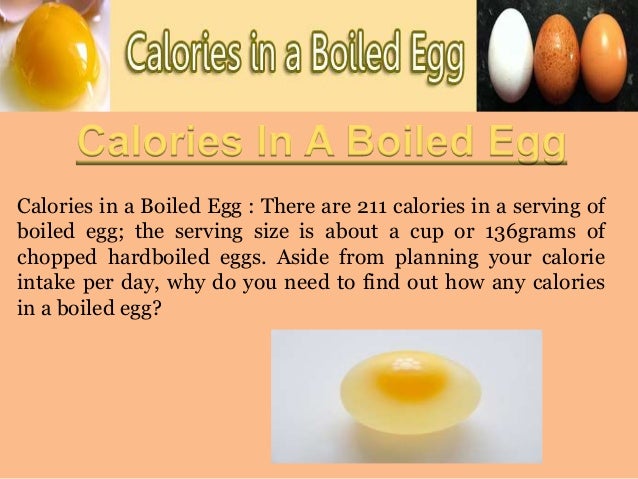The PowerPoint slide prominently displays nutritional information about boiled eggs. In the top left corner, there is a detailed image of a boiled egg with the yolk clearly visible and a small portion of the white egg at the bottom. Adjacent to this, towards the right, a small photograph showcases three distinct eggs: one white, one dark with black freckles, and one yellow-brownish egg on a black surface. Centrally positioned, the title "Calories in a Boiled Egg" stands out in yellow font. Below this title, about three-fifths of the slide consists of a tan or light peach background where another title repeats "Calories in a Boiled Egg" in yellow with a darker yellow underline. Beneath this, a paragraph in dark blue or black font states, "There are 211 calories in a serving of boiled egg. The serving size is about a cup or 136 grams of chopped hard-boiled eggs. Aside from planning your calorie intake per day, why do you need to find out how many calories in a boiled egg?" Finally, at the bottom middle-right of the slide, there is an image of a boiled egg cut in half, showcasing the white exterior and vibrant yellow yolk against a white background.